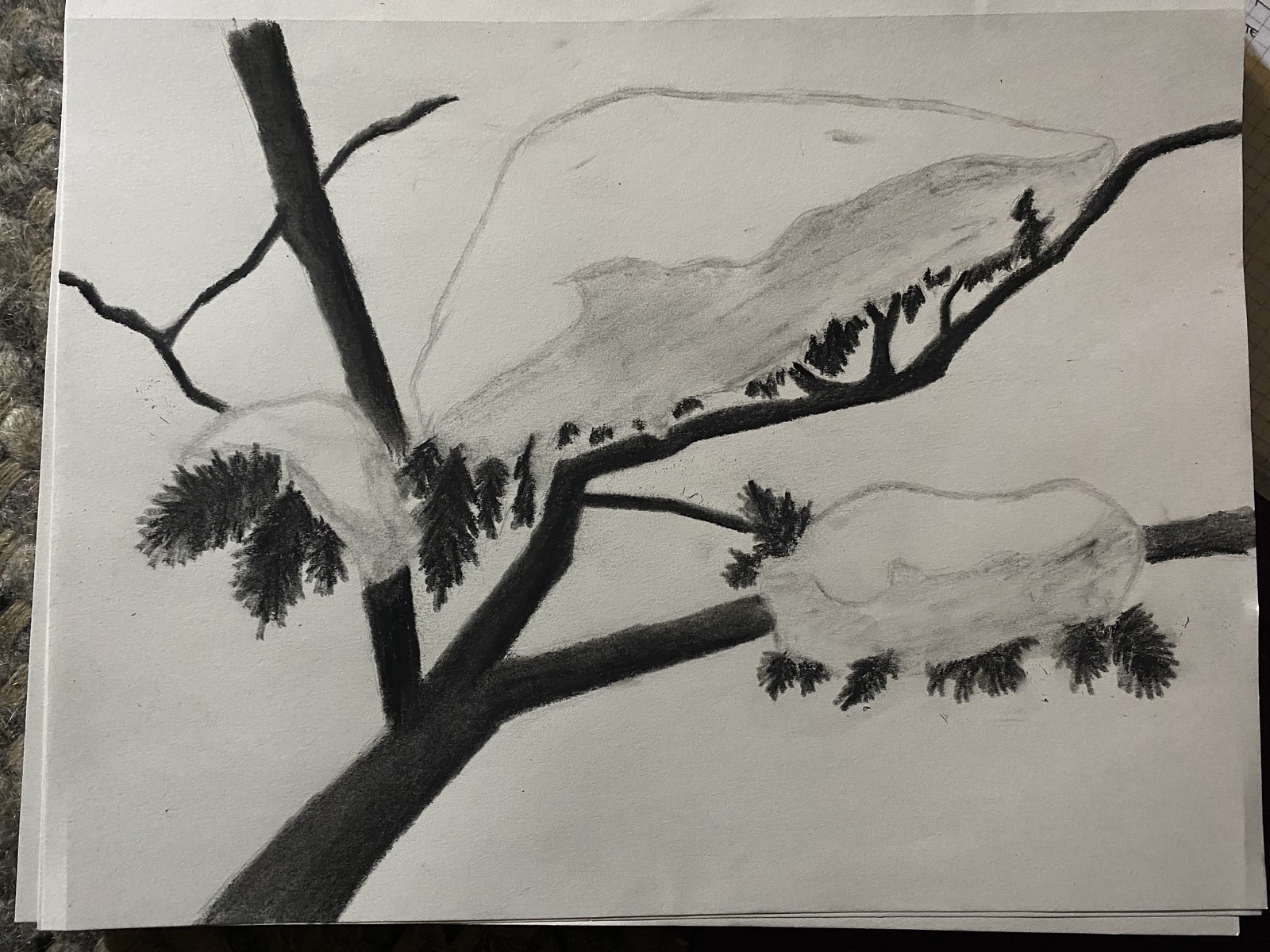This detailed pencil or monochromatic drawing, rendered in dark gray, brown, and black tones, is crafted on a piece of crisp white paper. Beneath this main artwork, a few additional sheets are subtly visible, suggesting a layered arrangement on a flat surface. To the right side of the composition, we observe a gridded structure that hints at the setting likely being a desk or workspace.

The artwork itself intricately depicts a tree branch, specifically resembling that of a pine tree, characterized by needle-like leaves. The primary subject is composed of three significant branches, each adorned with clusters of needles, all blanketed under a thick layer of snow, delicately captured in monochrome hues. Contrasting this, other visible branches in the drawing are bare, devoid of foliage, and not cloaked in snow, which highlights the stark beauty of the snow-laden pine branches. This captivating artwork seamlessly merges meticulous detail with the serene simplicity of winter's embrace.